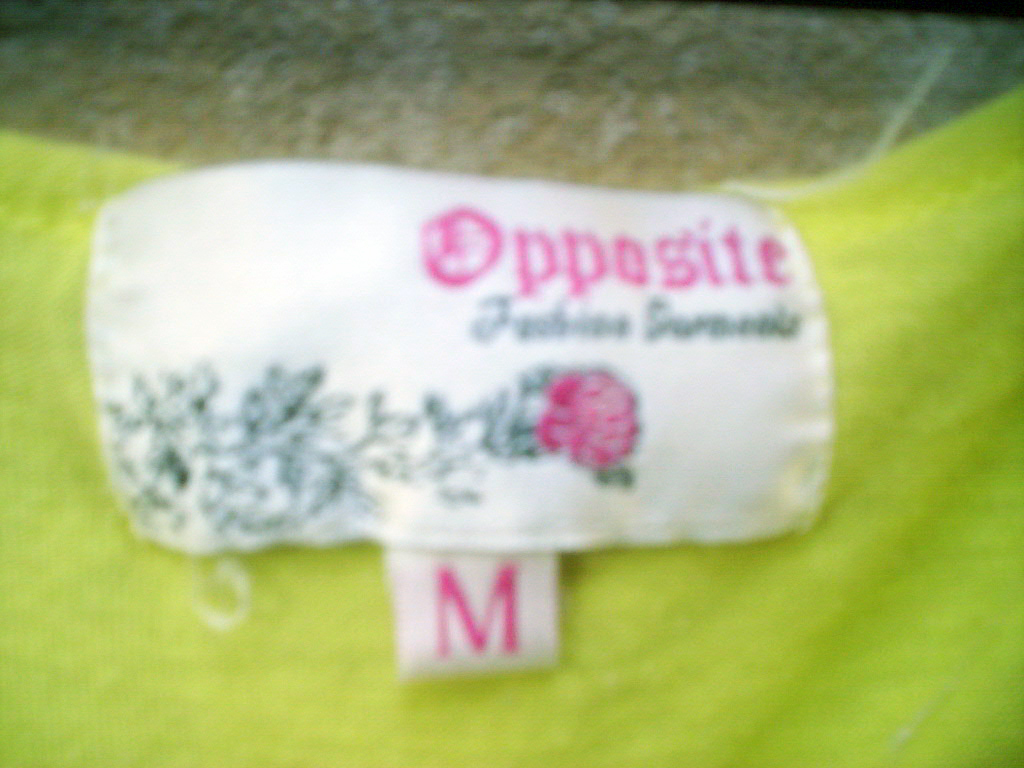This is a close-up photograph of a tag sewn onto the back of a bright lime green shirt, set against a speckled tan and brown background, possibly a tabletop. The tag is white and rectangular, adorned with a floral design featuring green leaves on the bottom left and a pink rose extending to the right. At the top right corner of the tag, the word "Opposite" is written in a black, gothic font. Below that, in black cursive script, it says "fashion," although the next word is unreadable due to the blurriness of the image. Attached beneath this main tag is a smaller white tag displaying a capital "M" in pink, indicating the shirt size as medium. The tags are sewn on the shirt's fabric, which appears only partially in the image.